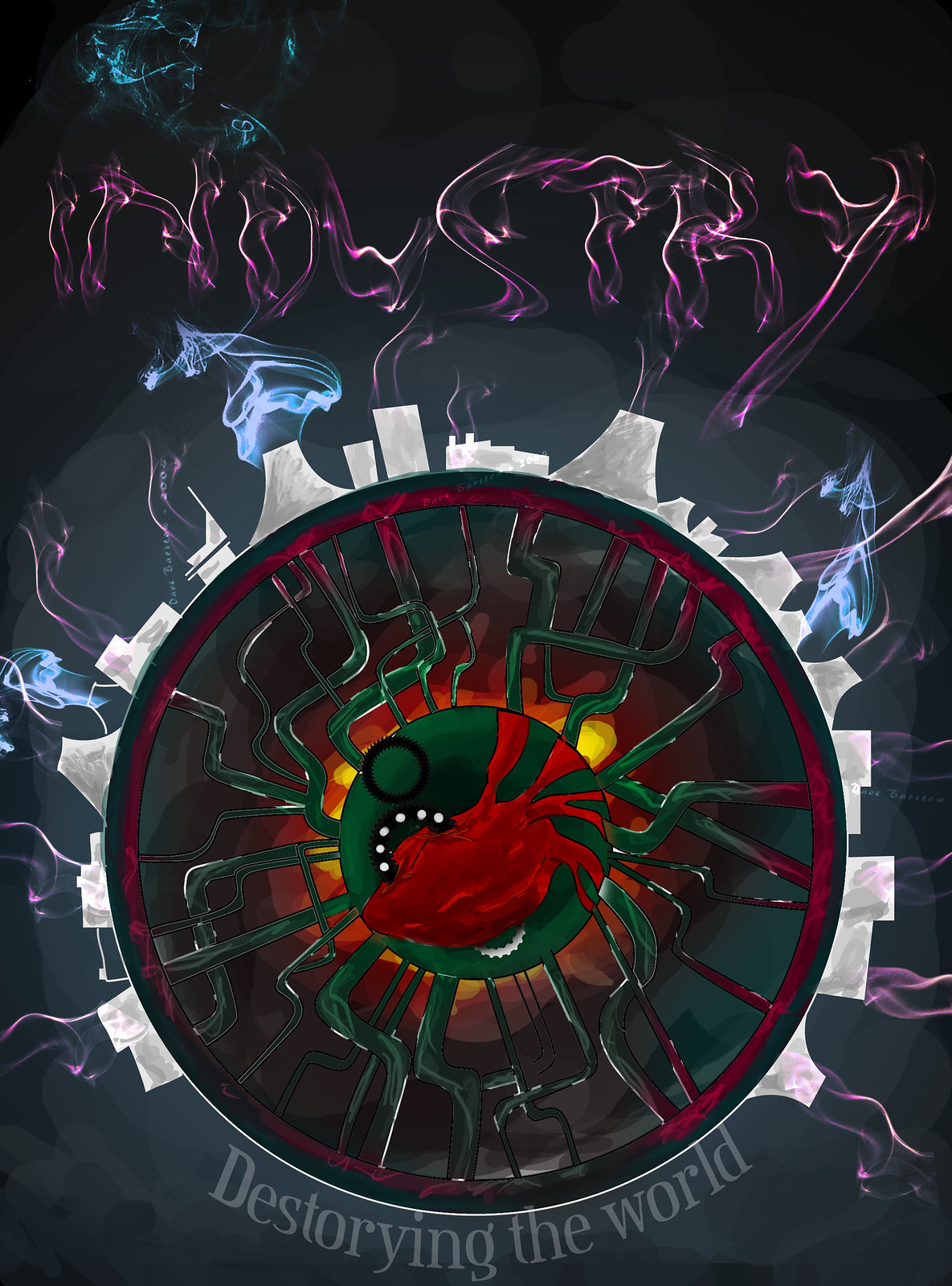The image, which seems to be an artistic, abstract representation suitable for an album cover, features a central red anatomical heart encased within a green circle. This heart is connected to a web of green pipes extending outward to a larger encompassing circle. Surrounding this larger circle are white factory smokestacks, arranged primarily from the lower right to the lower left, emitting swirling clouds of pink, blue, and purple smoke. The background of the image is predominantly black and gray, adding a contrast to the vivid central elements. At the top of the image, the word "Industry" is inscribed in a smoky, wavy purple font, as if formed by rising smoke. Below the heart and circles, the text "Destroying the World" is prominently displayed, tying together the visual theme that suggests a critique of industrial impacts on the planet.